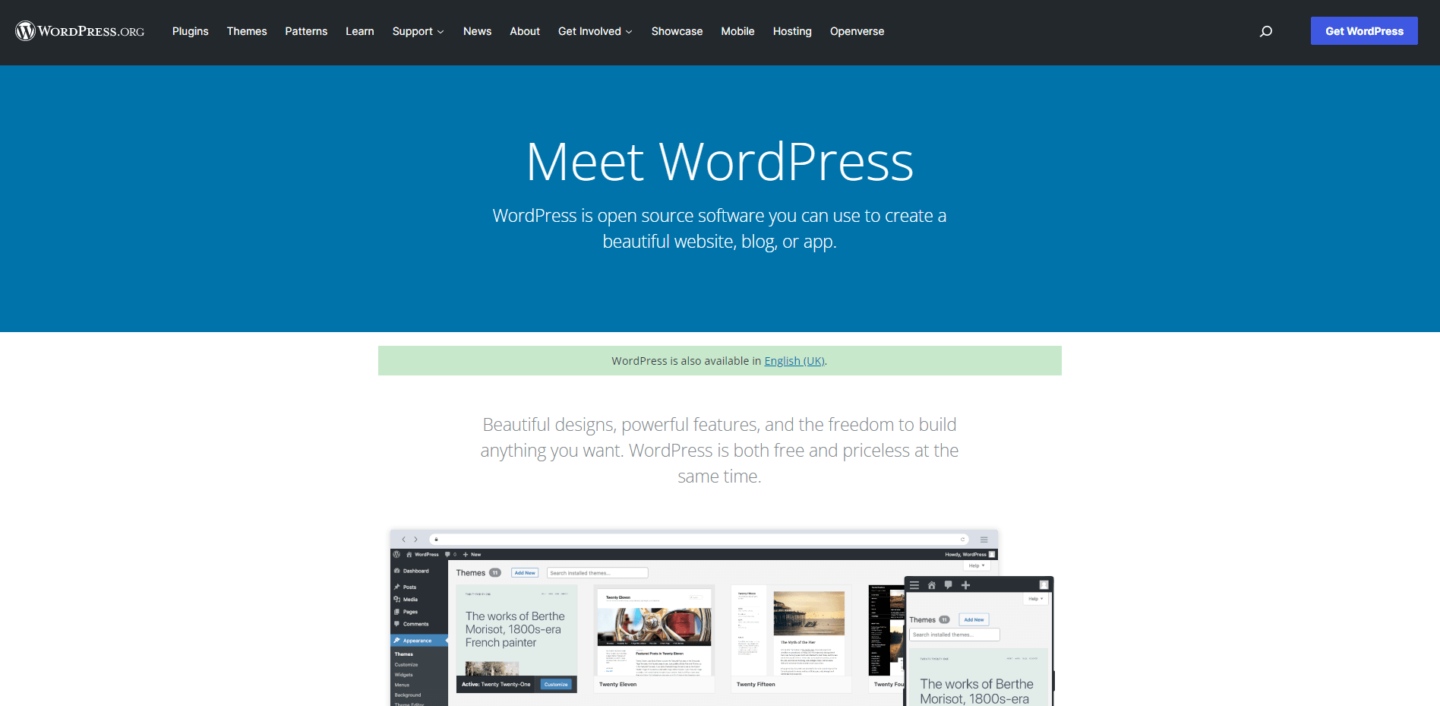This image is a detailed screenshot of the WordPress.org website. At the top left of the screen, the header features the WordPress logo, a 'W' inside a white circle, followed by the site name 'wordpress.org.' The black header bar contains various navigation options listed from left to right: Plugins, Themes, Patterns, Learn, Support, News, About, Get Involved, Showcase, Mobile, Hosting, and Openverse. On the top right corner, there is a blue button labeled 'Get WordPress.'

Directly beneath the header is a prominent blue banner with white text stating, "Meet WordPress. WordPress is open-source software you can use to create a beautiful website, blog, or app." Below the banner, additional text reads, "WordPress is also available in English (UK). Beautiful designs, powerful features, and the freedom to build anything you want. WordPress is both free and priceless at the same time."

Further down in the image, there are several smaller images displaying different website designs, hinting at what can be achieved using WordPress. On the left side of the screen, there's a black navigation bar providing additional links and options for site visitors.